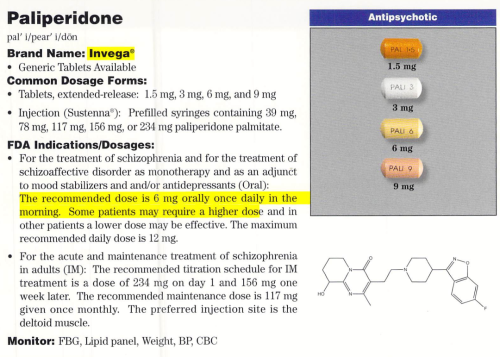This image features various forms of the antipsychotic medication known as Paliperidone, marketed under the brand name Invega and available in generic formulations. The picture displays the medication in different colored tablets — orange, white, yellow, and orangey tan. It provides detailed information on FDA indications, dosages, and treatment protocols.

### Indications and Uses:
- **Treatment of Schizophrenia**: Paliperidone is used for the treatment of schizophrenia.
- **Schizoaffective Disorder**: Effective as monotherapy or as an adjunct to mood stabilizers and/or antidepressants.

### Dosage Information:
- **Oral Tablets**:
  - **Common Dosage**: The recommended dose is 6 milligrams taken orally once daily in the morning.
  - **Range**: Some patients may need a higher dose, while others may find a lower dose effective. The maximum daily dose is 12 milligrams.

- **Injectable Form**:
  - For the acute and maintenance treatment of schizophrenia in adults:
    - **Initial Dosing Schedule**: 234 milligrams on day one, followed by 156 milligrams one week later.
    - **Maintenance Dosing**: 117 milligrams administered once monthly.
    - **Preferred Injection Site**: Deltoid muscle.

### Monitoring:
Highlighted under monitoring guidelines are the following parameters which should be assessed regularly:
- **FBG (Fasting Blood Glucose)**
- **Lipid Panel**
- **Weight**
- **Blood Pressure (BP)**
- **Complete Blood Count (CBC)**

These guidelines and information are crucial for ensuring the effective and safe use of Paliperidone in the treatment of relevant psychiatric conditions.